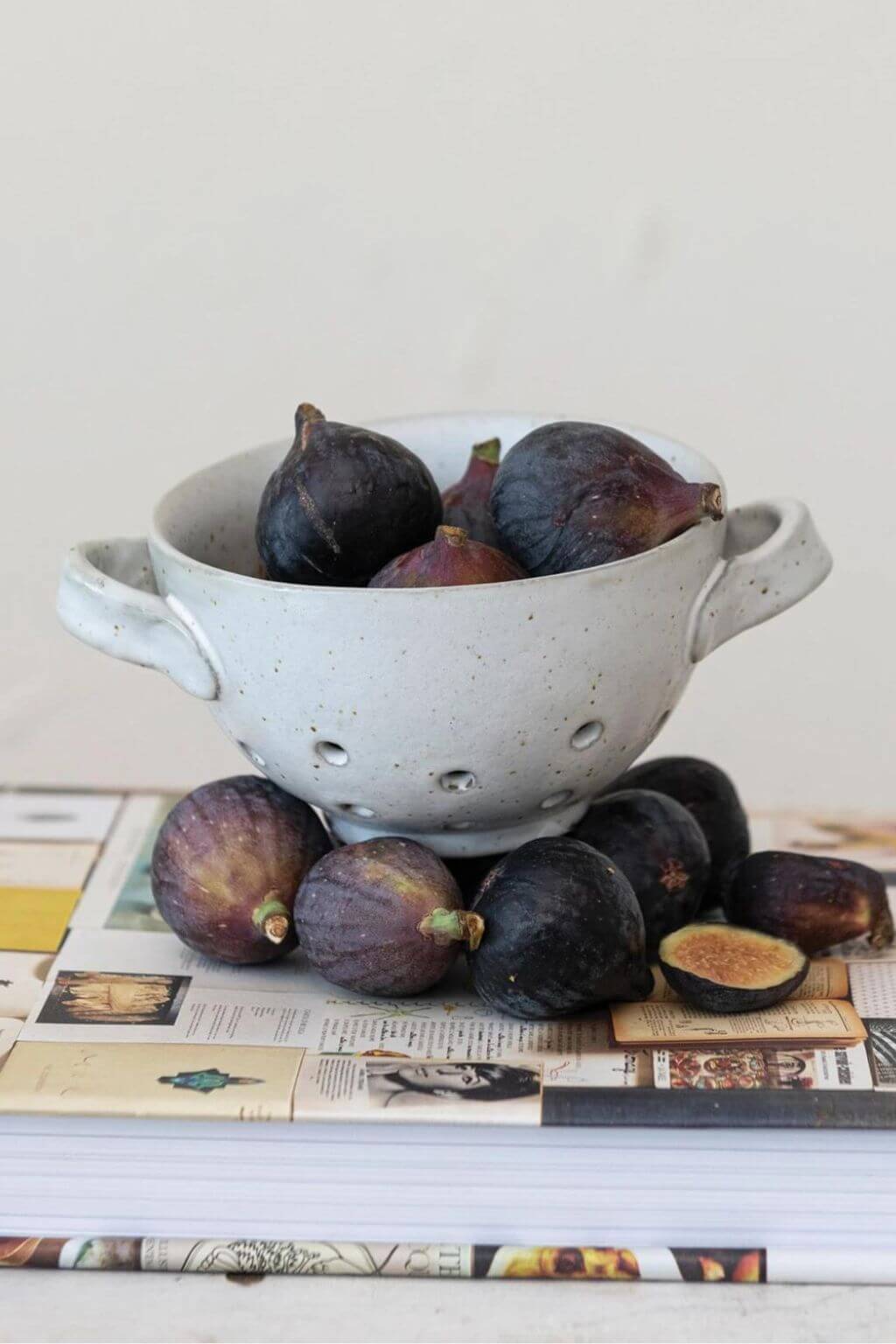The photograph captures a scene set against a clean, white background, featuring a white colander with drainage holes in the bottom and handles on either side. The colander is filled with what appear to be freshly harvested onions, their green tops trimmed. Surrounding the colander on a surface that looks like it is covered with an old, multicolored book featuring various images, are several more onions, with one of them cut in half, revealing its layers. The book seems to be quite thick, approximately an inch to an inch and a half. Scattered around are some rolled-up papers, adding to the rustic, homey atmosphere. The onions in the colander and those around it form the focal point of the image, all set against a stark white wall in the background.